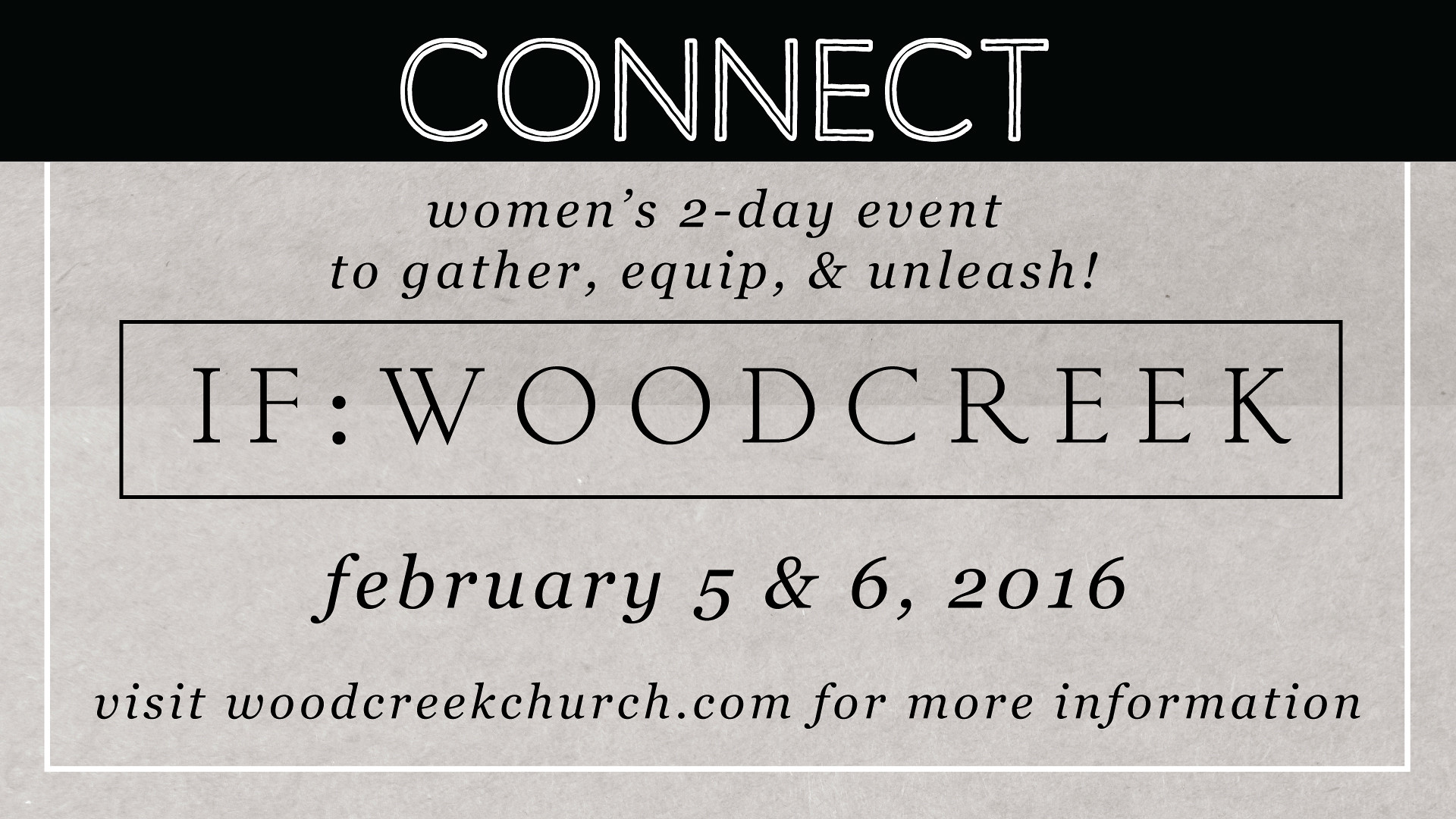This image, designed as a social media banner for an upcoming event, features a horizontally aligned rectangular format with a gray recycled-paper-like background. A black bar spans the top of the graphic, centered within it is the word "CONNECT" in white letters, each with a line of black through them. Directly below, on the gray background, is the phrase "to gather, equip, and unleash!" 

The main section of the graphic highlights a "Women's 2-Day Event." Below this, enclosed in a small rectangular box bordered in black, are the words "IF: WOOD CREEK" in all-caps. Following this, the dates of the event, "February 5 and 6, 2016," are noted along with a call to action: "Visit woodcreekchurch.com for more information." The bottom and sides of the main text area are bordered by a white line, but the top remains open where it meets the black "CONNECT" bar.